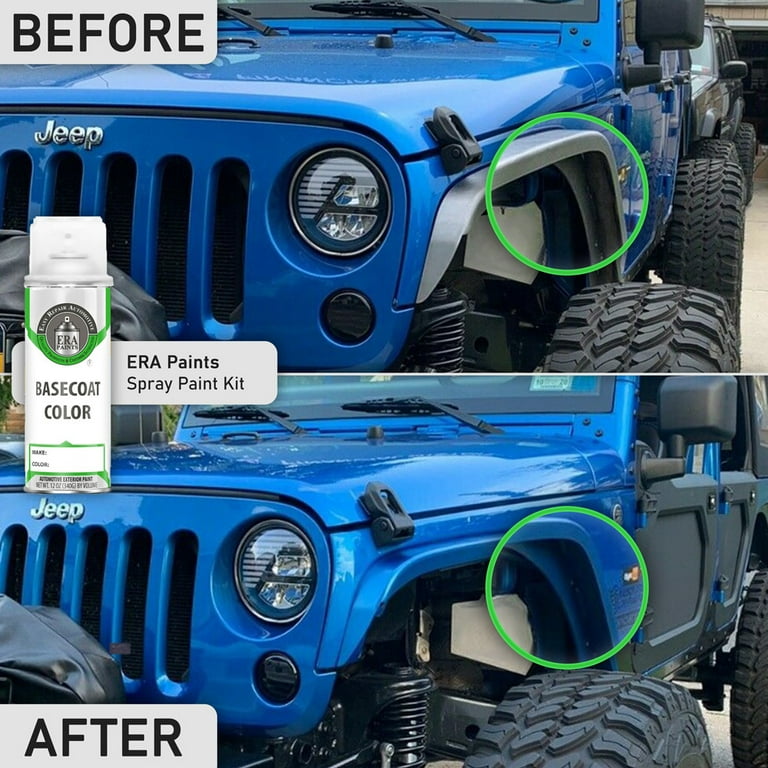Here's the cleaned-up and detailed caption:

This advertisement image is divided into two stacked photographs, each taken outdoors, and illustrates a before-and-after transformation of a Jeep using the ERA Paint Spray Paint Kit. The square image measures approximately six inches by six inches. The top photograph, labeled "Before" in the upper left corner with black text on a gray background, shows the front end of a blue Jeep. The Jeep's grille features the silver "Jeep" logo, and several black elements, including the windshield frame, wipers, and mirrors, are visible. A gray wheel well on the driver's side front tire is highlighted with a green circle outline.

The bottom photograph, labeled "After" in the lower left corner with black text on a gray background, is identical except for the transformation: the previously gray wheel well is now painted blue to match the rest of the Jeep. 

Between the two photographs, on the left side, is a white spray paint can labeled "Base Coat Color," alongside a white box that reads "ERA Paint Spray Paint Kit" in black text. The can has a black top and is highlighted with a circle featuring a design with gray and green sections. The advertisement effectively showcases the product's ability to seamlessly color-match and upgrade the Jeep's appearance.